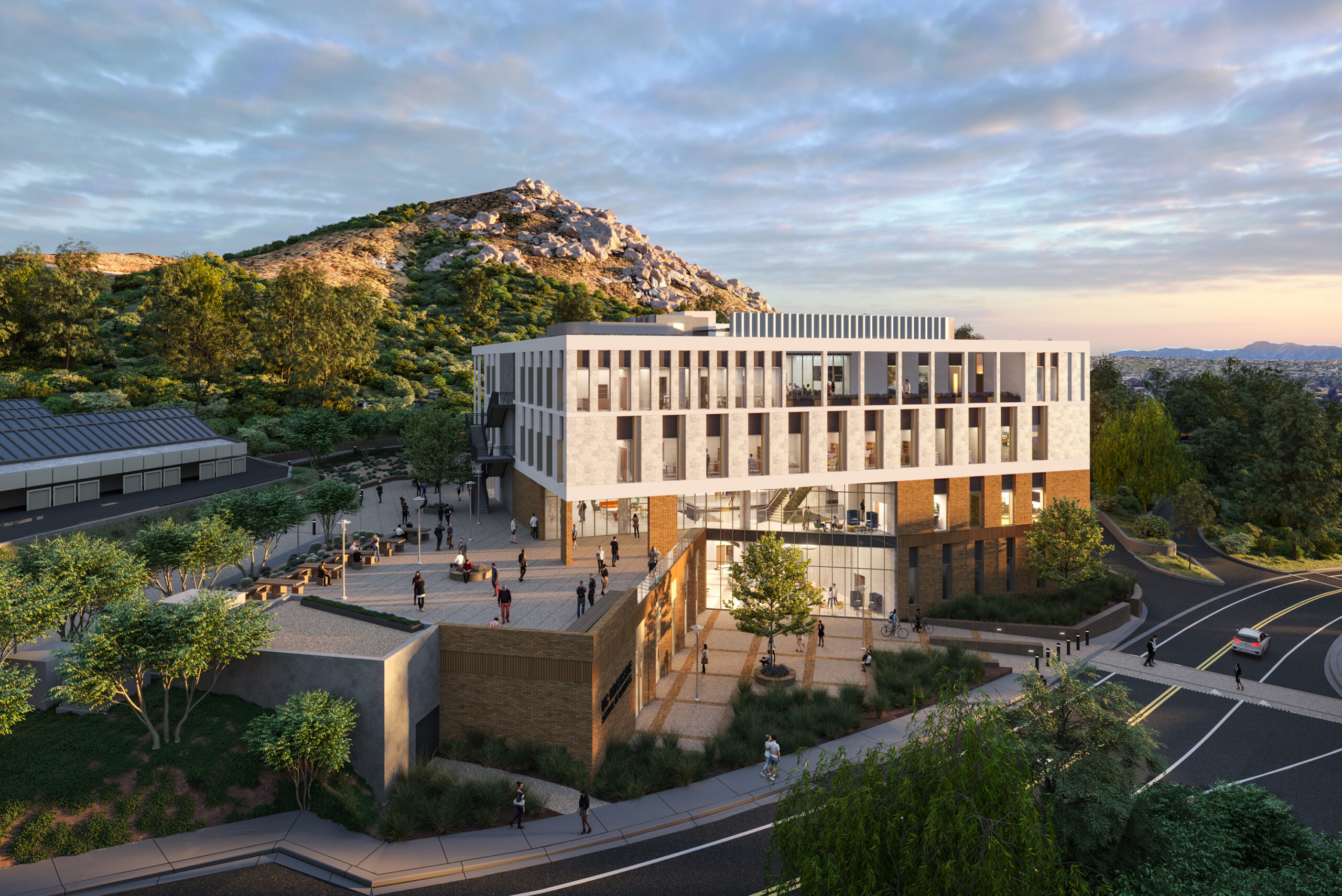This photograph, taken from an elevated angle, captures a large multi-story building, reminiscent of a college campus, surrounded by a vivid landscape of green trees and mountains. The building itself features a mix of brownish and grayish brick materials, with two distinct sections: one with four floors and another single-floor section that includes a platform where people can gather. The rooftop and glass entranceway suggest bustling activity, likely of students. Numerous tall, rectangular windows punctuate the building’s angular façade. In the foreground, an asphalt road with a single car driving away intersects with sidewalks and crosswalks, where several people can be seen walking. The scene is set against a backdrop of a large, tree-covered mountain with rocky, barren peaks. Above, the sky is dotted with wispy white and gray clouds, indicating a sunny day with intermittent cloud cover. The abundance of greenery suggests the season is either spring or early fall.